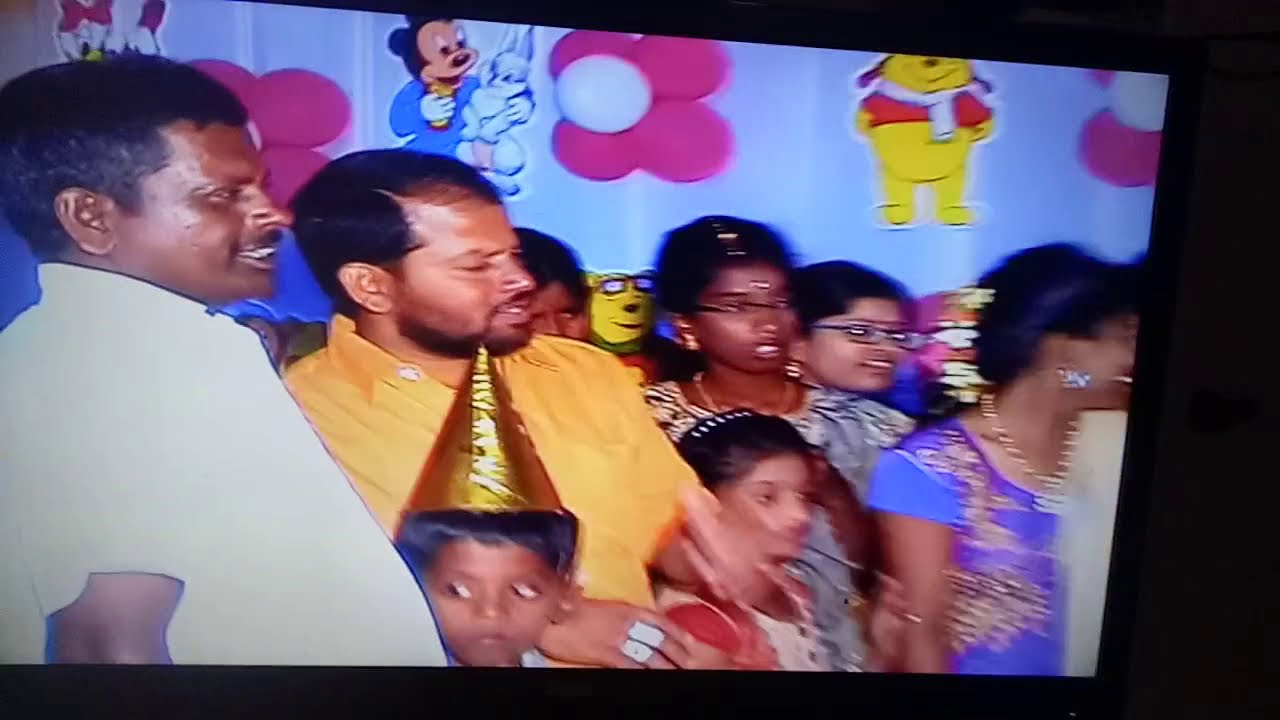The photograph shows a slightly angled and blurry snapshot of a TV screen displaying a family gathering. The setting appears to be an Indian or Middle Eastern celebration, potentially a child's birthday party, as indicated by the young boy wearing a gold birthday hat. The family, comprising three adult males, three adult females, and two children, is adorned in vibrant, ornate attire with intricate embroidery and fine jewelry. They stand against a light pink wall decorated with several Disney character decals, including an aviator Winnie the Pooh in a red shirt, a musician Winnie the Pooh, Mickey Mouse in a blue robe holding a white rabbit, and the top of Daisy Duck. The wall also features decorative elements such as pink flowers and blue moons with white centers. The picture itself is of poor quality, taken from an angle, and partly obscured by the photographer.